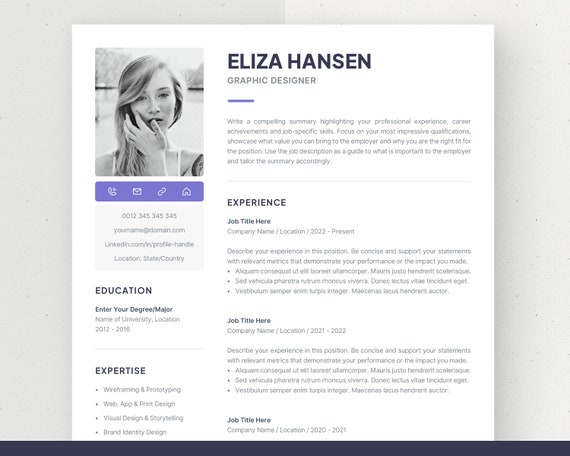The image is a resume belonging to Eliza Hansen, a graphic designer. It is presented on a plain white piece of paper featuring a clean and straightforward template with black text and subtle purple accents. In the top left corner, there's a black and white photograph of Eliza, a woman with her hand across her face, which provides a personal touch. Below the photo, her contact information is neatly listed with icons representing a phone, email, LinkedIn, and location, all in purple. The left column includes her education details, summarizing her degree, major, and the duration at her university, followed by a section highlighting her expertise with bullet points that outline her skills. The main body of the resume prominently displays her name, "Eliza Hansen," with the title "Graphic Designer" beneath it, underlined by a thin purple line. The right column contains a brief summary of her skills and elaborates on her professional experience, listing job titles, company names, locations, and the duration of employment, plus space to describe her roles and accomplishments. The overall design is simple yet effective, ensuring all critical information is easily accessible.